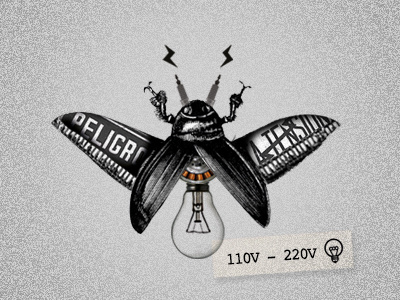The image depicts a creatively illustrated beetle or insect, centrally positioned on a white and black speckled surface, resembling a piece of artwork or a pin. The beetle, primarily black with intricate silver engravings and lettering, features its wings open. Beneath the wings is an unlit light bulb where the abdomen would typically be, symbolizing some form of electrical or light-related symbolism. The insect has two distinct antennae with black lightning bolt designs emanating from them, and it possesses claw-like appendages positioned near its head. Additional details include smaller airplane-like wings with partial and unclear silver inscriptions, such as "E-L-I-G-R." At the bottom of the image, a tag reads "110V-220V," accompanied by another light bulb symbol, suggesting an electrical theme. The overall artwork merges organic beetle characteristics with electrical motifs, primarily rendered in black and white, aside from some small copper details.